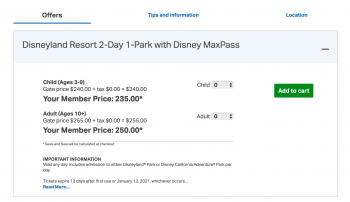The image is a low-quality, cropped screenshot taken from a website, featuring a somewhat blurry and text-heavy interface. The screenshot highlights the "Offers" section in the top navigation bar with a blue underline. Adjacent to this section are "Tips and Information" and "Location" tabs. 

Below the navigation, there is a primary content box titled "Disneyland Resort Two-Day One Park with Disney Max Pass." The box lists ticket pricing, including a children's ticket at a member price of $235 and an adult ticket at a member price of $250. Underneath the pricing, there is a quantity selector that is currently set to zero, allowing users to choose the number of tickets they wish to purchase. At the bottom of the box, there is a prominent green "Add to Cart" button.